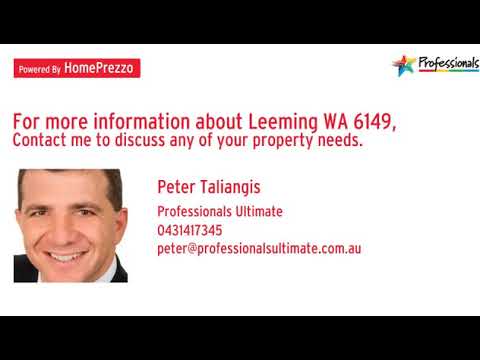This image is a rectangular, color business card with a landscape orientation, featured within a thick black border at the top and bottom. The card is predominantly white with red and black text. In the top left corner, a red rectangle with white letters reads, "Powered by Home Prezzo." Opposite that, in the top right corner, the word "Professionals" appears, accompanied by a rainbow star and a rainbow underline. Below these elements, and starting from the left side, a red-font sentence reads, "For more information about Leeming WA 6149, contact me to discuss any of your property needs." Adjacent to this text, on the left side, is a portrait of a middle-aged, clean-shaven man in a business suit and white shirt, smiling at the camera. To the right of his photo, the text in red identifies him as "Peter Talliangas," followed by "Professionals Ultimate," his phone number "0431 417 345," and his email "peter@professionalsultimate.com.au."